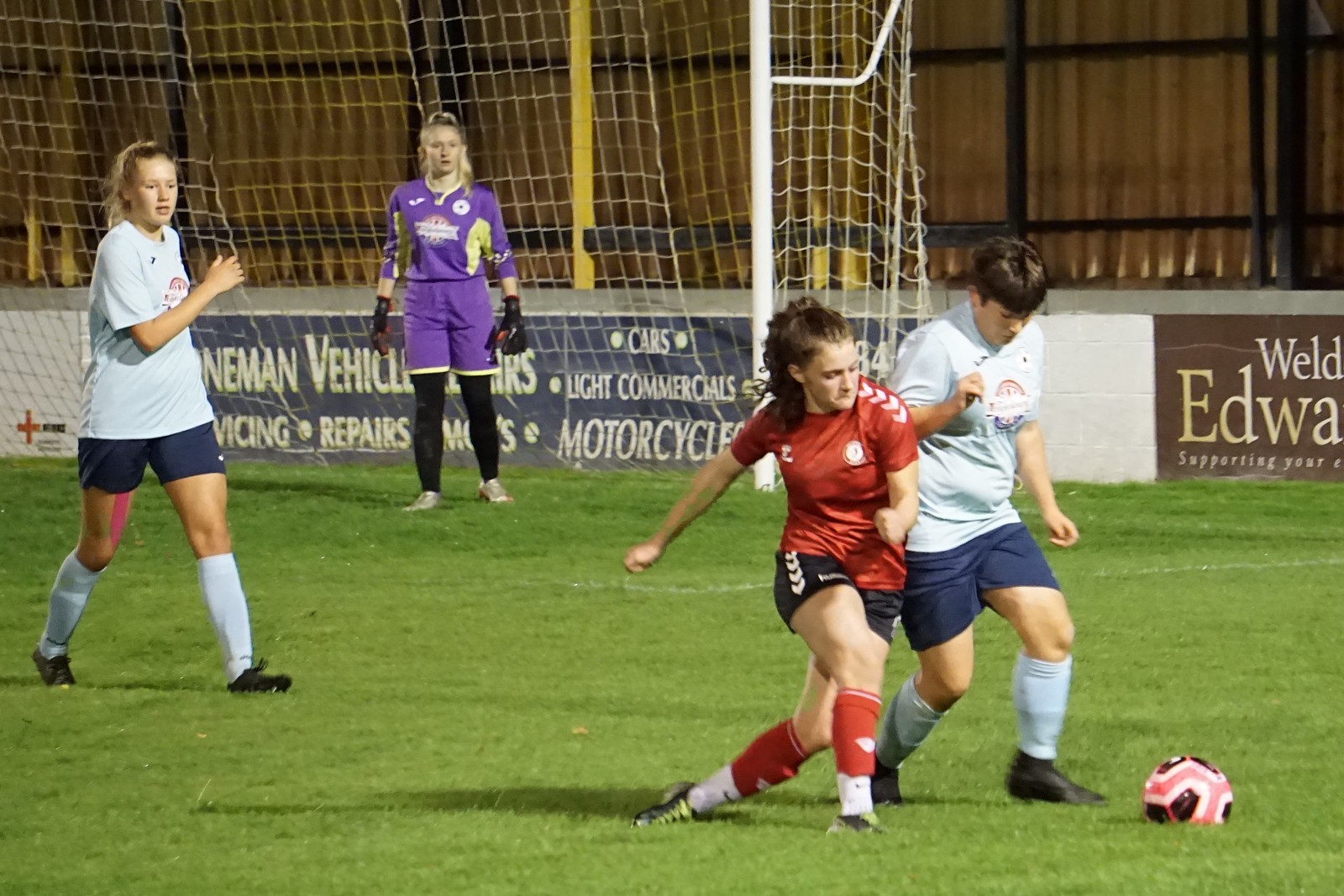The image depicts a lively soccer game set on a vibrant green field under a clear sky. Four players are captured in action. In the foreground, a female player with brown hair tied back in a ponytail, dressed in a red jersey, red socks, and black shorts, is lunging towards the ball alongside a male player in a light blue t-shirt, dark blue shorts, and tall white socks. The soccer ball, which is a mix of pink, black, and white, lies between them on the grass. 

To the left, a female player in a white t-shirt with navy blue shorts and tall white socks is seen running towards the duo, adding to the intensity of the moment. In the background, centered in front of a large white soccer net, stands the goalie, a blonde girl wearing a purple top, purple shorts, and black leggings. She has her hair pulled back into a ponytail and is also adorned with black gloves.

Beyond the net, a low fence lined with partially obscured banners bearing sponsor names can be seen, hinting at phrases like "cars," "light commercials," and "motorcycles." The setting indicates a bright, sunny day, and the overall scene captures the dynamic and engaging spirit of the soccer game.